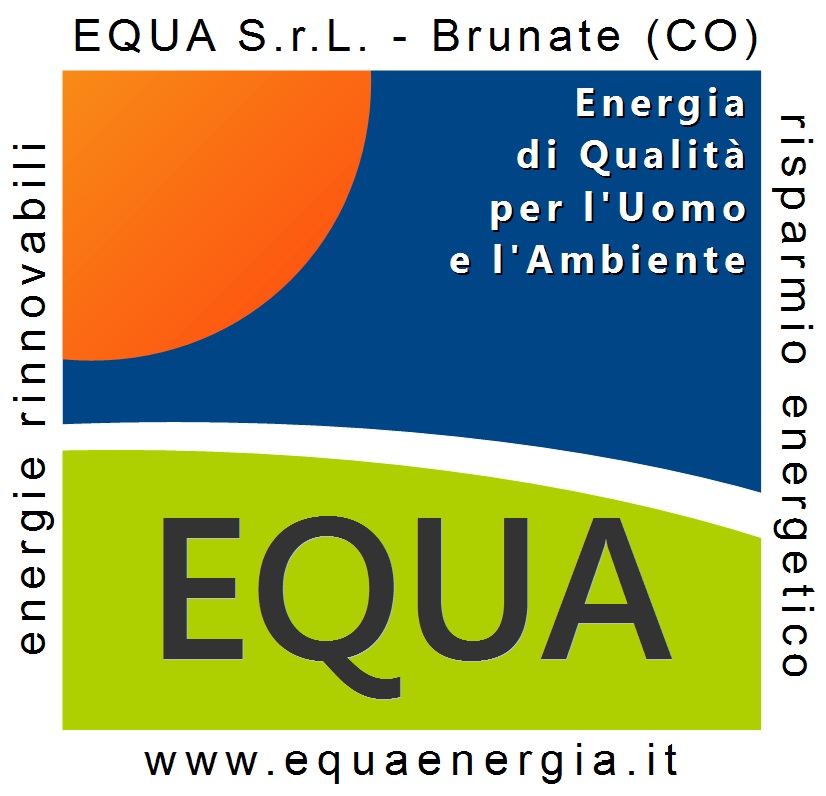The image features a prominently centered company logo styled with a blend of graphic design elements, suggesting it is an advertisement or a corporate emblem. The text is predominantly in Italian, enveloped within a square border, and includes words like "ENERGY," "RINOVABILI," "AQUA SRL BRUNATE," "RISPARMIO ENERGETICO," and the website "www.equaenergia.it." The logo itself is characterized by vibrant colors, with a spearmint green lower section and a navy blue upper section, separated by a curved white stripe. The upper-left corner showcases an orange half-circle resembling a sun. The logo's central part features additional Italian text—"ENERGIA DI QUALITÀ PER L'UOMO E L'AMBIENTE"—and the company name "EQUA" in uppercase gray lettering. The color palette includes orange, blue, white, green, and black, ensuring a visually cohesive and professional appearance.